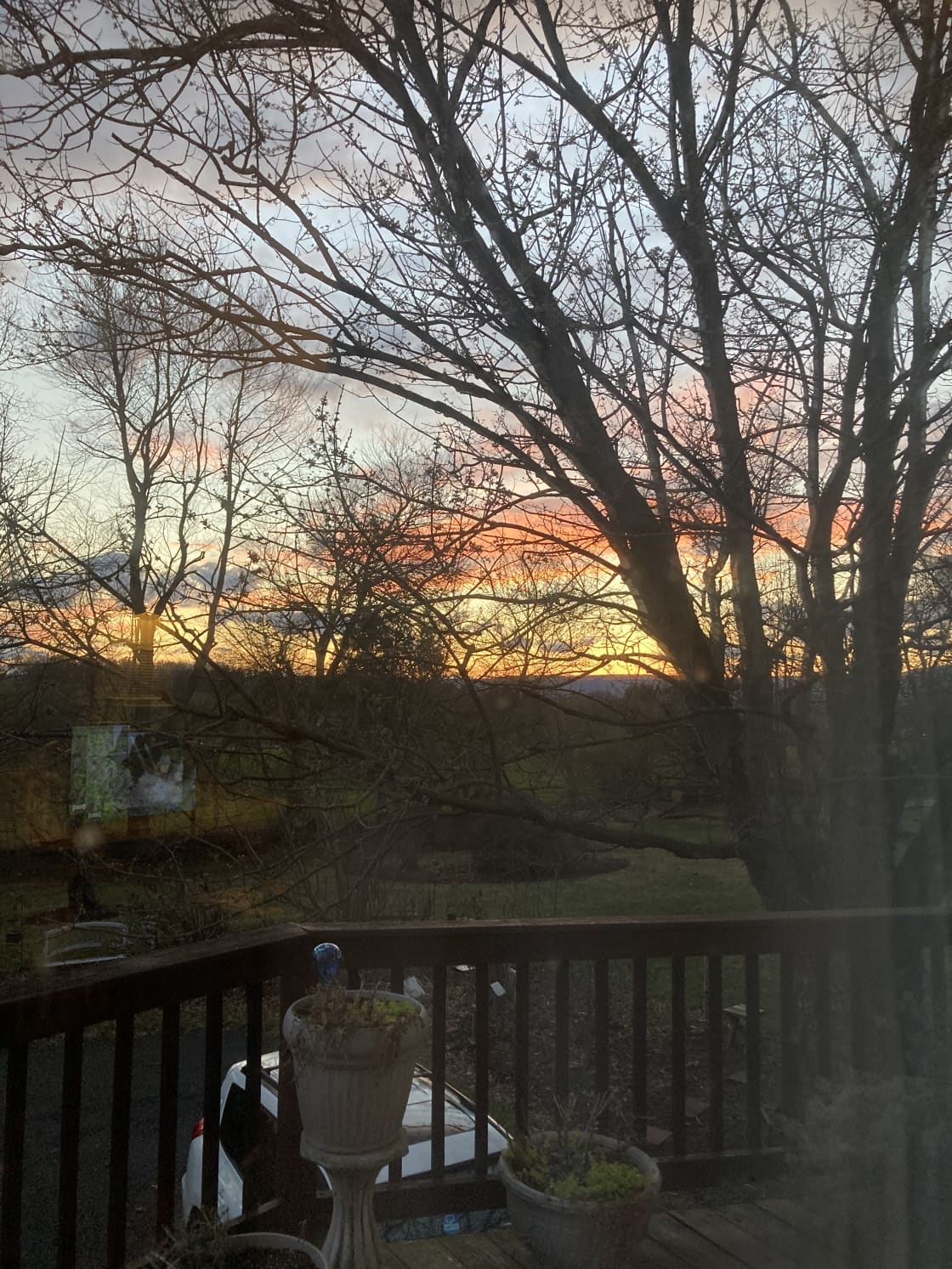The photograph captures a serene sunset scene from what appears to be a residential deck or porch. The vantage point looks out over a grassy backyard dotted with leafless trees, hinting at a fall setting. Dominating the right side of the image is a very tall tree with sprawling branches that reach leftward across the frame. The wooden deck's railing runs horizontally across the bottom quarter of the image, bending slightly leftward about one-fifth of the way up from the bottom. This railing frames the scene and is topped with wooden rails. Directly in front of the railing, two to three light gray ceramic planters, some containing partially alive foliage, sit on the deck floor. 

Below the deck, the top rear portion of a white car or SUV is visible in the driveway. The sky along the horizon, which bisects the image, features a sunset with a gradient of golden yellow near the horizon, transitioning to soft pinks and deeper reddish clouds, capped by a light blue sky. The entire foreground appears somewhat dark, possibly due to dusk lighting conditions or the quality of the photograph. Overall, the image conveys a peaceful, late-afternoon moment with the striking backdrop of a colorful sunset.